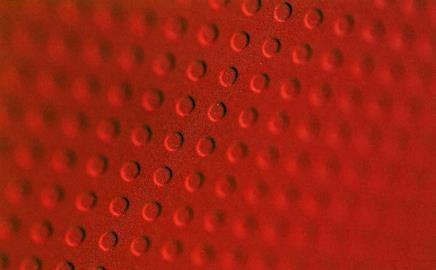This color photograph, captured in a landscape orientation, features a red textured surface with a grid of small, pea-sized bumps. These bumps form a pattern of horizontal and vertical rows, creating approximately eight rows horizontally and fifteen rows vertically. Depending on the viewer's perspective, the bumps can appear as either raised protrusions or indents, contributing to an optical illusion. The central part of the image is in clear focus, showing crisp details of the bumps, while the upper left and lower right corners are blurred, giving a sense of depth and perspective shift. The overall style of the photograph is representational realism, emphasizing the intricate details and texture of the surface.